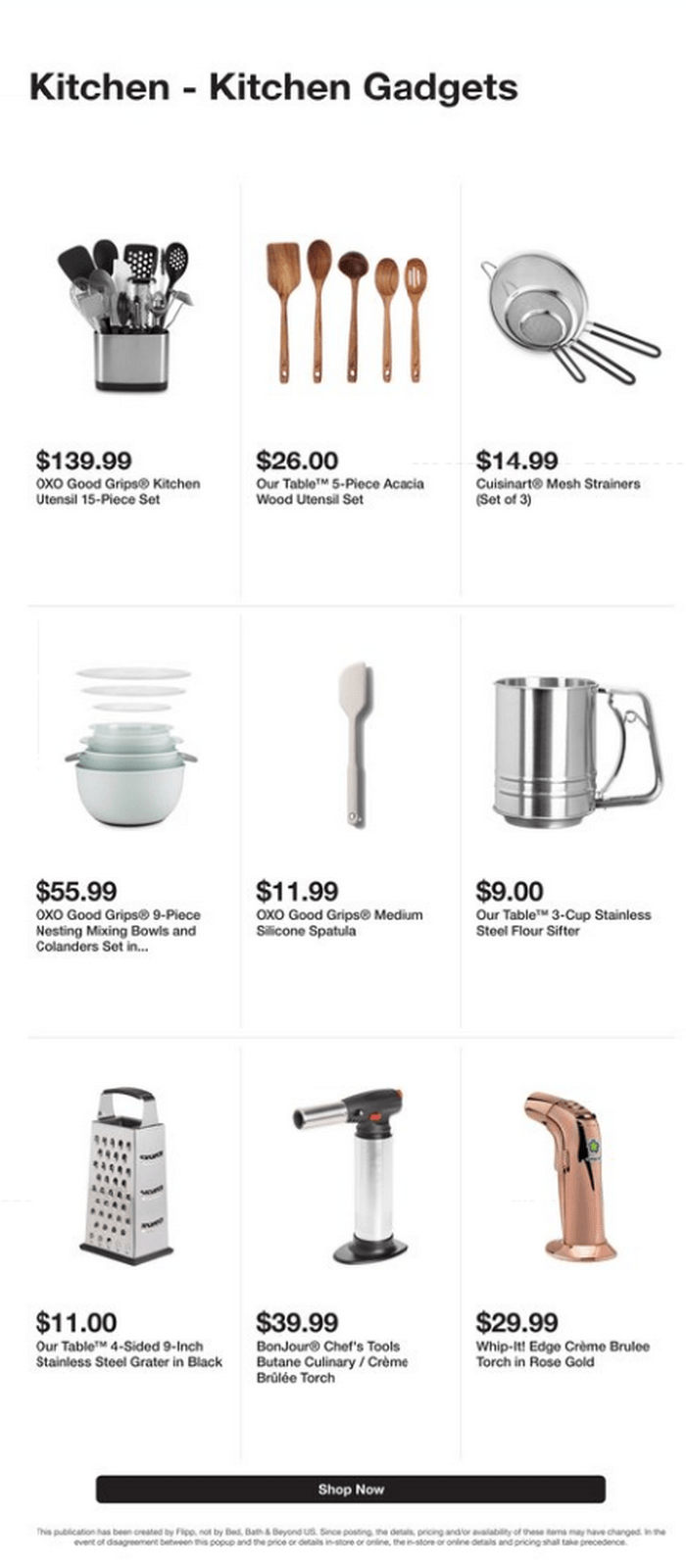In the top left corner of the image, a bold, rounded sans-serif font reads "Kitchen - Kitchen Gadgets." The image showcases several kitchen items. 

1. The first item is a metal canister with a black base and a black top, filled with various utensils including a black spatula, a black mixing spoon, a black slotted spatula, and a black skimmer. Below this, on the left, is the price in bold black letters: "$139.99." Directly beneath, in smaller, non-bold black text, it states "OXO® Good Grips Kitchen Utensil 15-Piece Set."

2. The second item consists of wooden utensils, including a spatula, a spoon, a ladle, another spoon, and a slotted spoon. The price, "$26.00," is displayed in bold black text underneath. In very small black sans-serif font, it reads "Our Table™ 5-Piece Acacia Wood Utensil Set."

3. To the right, three mesh strainers of varying sizes are arranged in descending order. They feature metal rims and black rubber handles. The price "$14.99" is displayed in bold black text below the strainers.